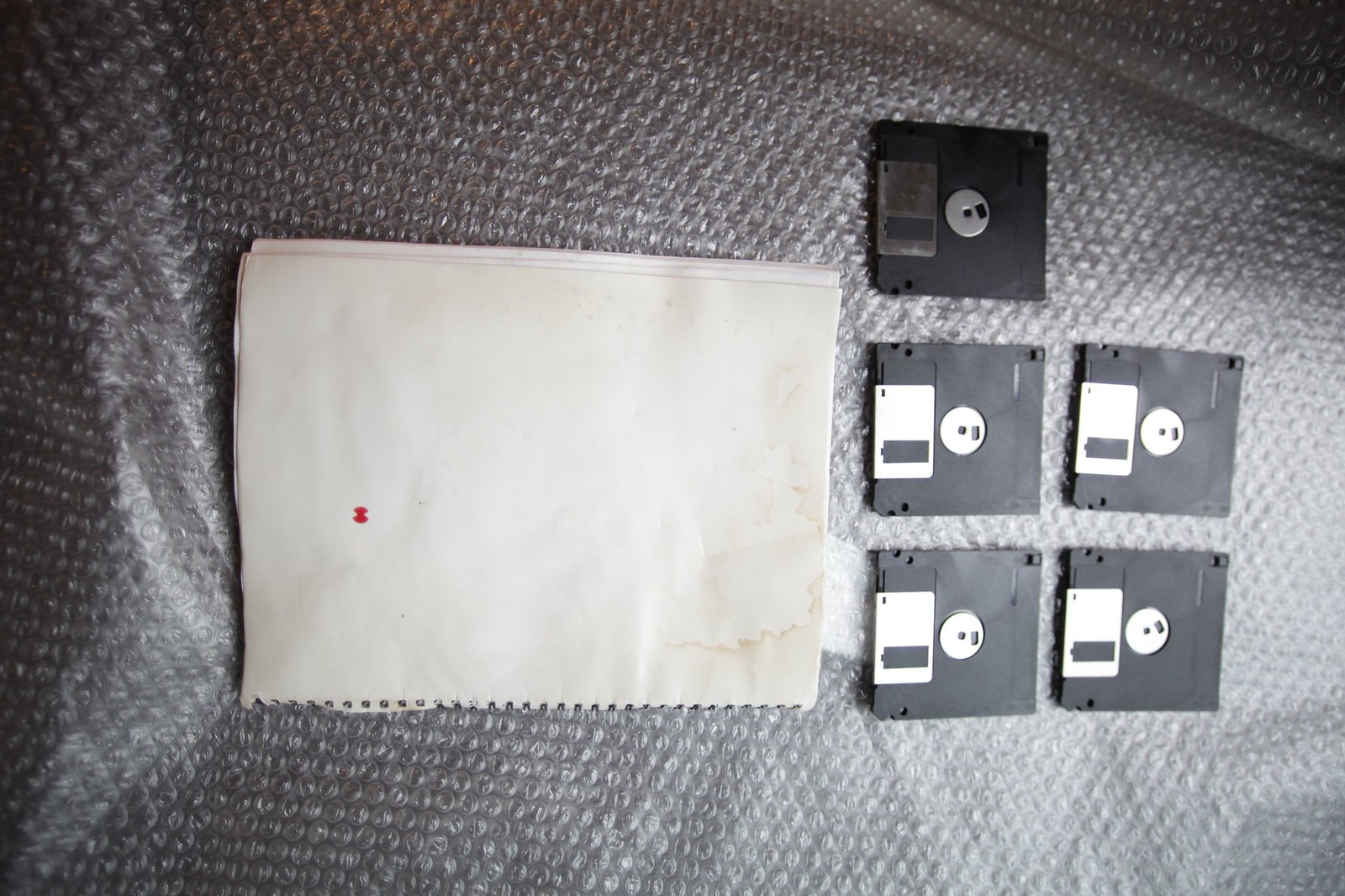This close-up image captures a collection of five black floppy disks and a worn sheet of white paper, all laid out on dark gray bubble wrap. The floppy disks are arranged neatly in two rows, with three in the top row and two in the bottom row. Each disk features a silver circle in the middle and a silver slot edge. To the left of the disks, the white paper, which appears to be torn from a spiral notebook, shows signs of heavy wear with wrinkles and water stains, possibly from coffee. The paper also has a tiny red dot and two light brown squiggly lines, suggesting further marks of age and use. The overall composition creates a juxtaposition between the dated technology of the floppy disks and the fragile, weathered state of the paper, all underlined by the textured gray bubble wrap beneath them.